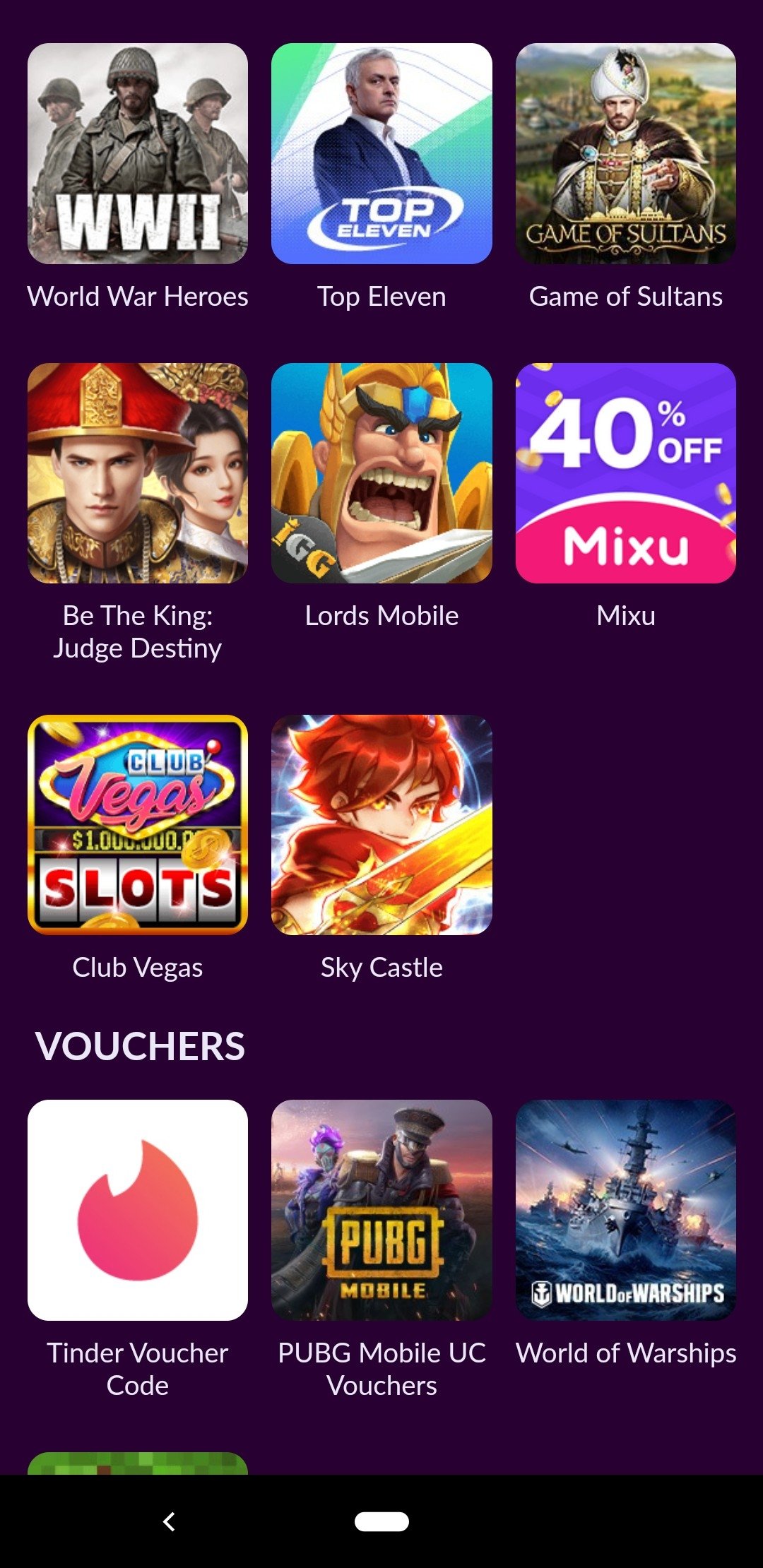Screenshot of a mobile application interface. The interface showcases various games and vouchers, organized into well-defined sections for easy navigation. Each game is highlighted with colorful icons and clear labels that capture the viewer's attention.

**Games featured:**
1. WW2 World War Heroes
2. Top Eleven
3. Games of Sultans
4. Be the King
5. Judge Destiny
6. Lords Mobile
7. Mixu
8. Club Vegas
9. Sky Castle

**Vouchers available:**
1. Tinder Voucher Code
2. PUBG Voucher
3. World of Warships Voucher
4. Minecraft Voucher

**Design details:**
The background of the interface is predominantly purple with a black bottom section. Despite being visually appealing, the functionality of the voucher system may be somewhat unclear. The overall layout is designed to be user-friendly, with distinct sections that make the navigation straightforward.